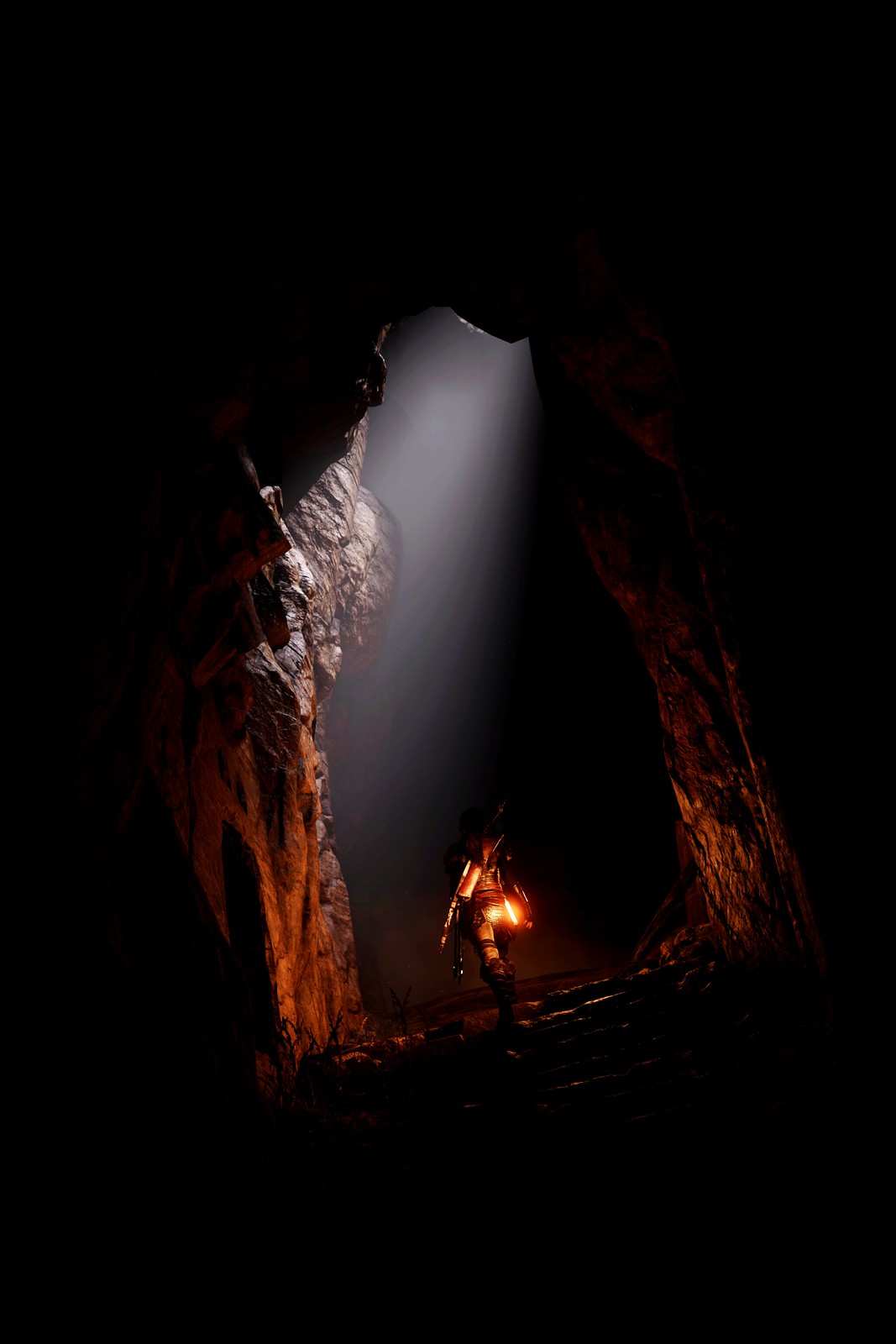The image depicts an AI-generated scene of a woman standing in the mouth of a cave, illuminated by a bright, white spotlight from above. The spotlight highlights the craggy, textured rocks of the cave, contrasting against the jet-black, featureless background that envelops the scene. The cave's opening is large, with the light revealing gradients of gray and reddish-brown rocks. The woman, identifiable by her silhouette, wears high boots and appears to carry a glowing object on her back. Details of her attire and hair color remain indistinguishable due to the intense and focused lighting. The scene evokes a mysterious atmosphere, with the character resembling a figure from a science-fiction narrative.